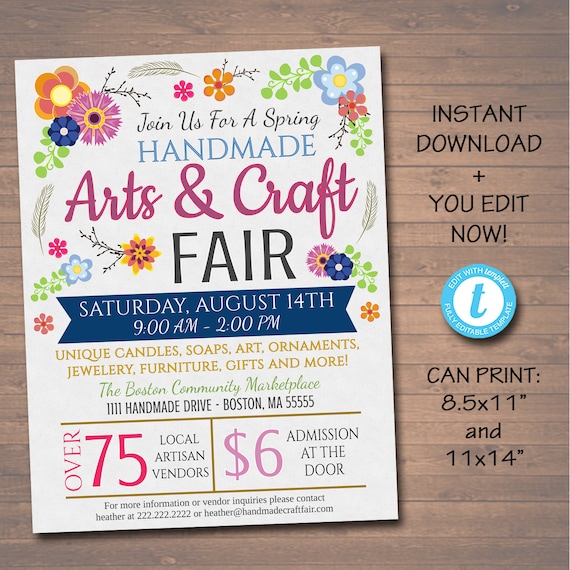The photograph showcases a vividly designed advertisement flyer for an app tailored for fair events, set against a rustic, light brown wooden background. On the right side of the flyer, bold black text announces "instant download, plus you edit now," followed by details in a circular light teal emblem featuring a prominent "T." It specifies printable formats as 8x5, 8.5x11, and 8x14 inches. The focal point is an elegantly sloped white card adorned with colorful flowers—blue, orange, and purple—with lush green leaves framing the corners. Centralized text in black declares, "Join us for a spring," with "handmade" highlighted in blue, followed by "arts and crafts fair" in cursive purple and "fair" again in black. A yellow banner ribbon prominently displays the event date and time: "Saturday, August 14th, 9 am to 2 pm." The flyer further mentions, "over 75 local and artisan vendors," and entrance details, "6 dollar admission at the door," with additional information summarized in fine black text at the bottom.